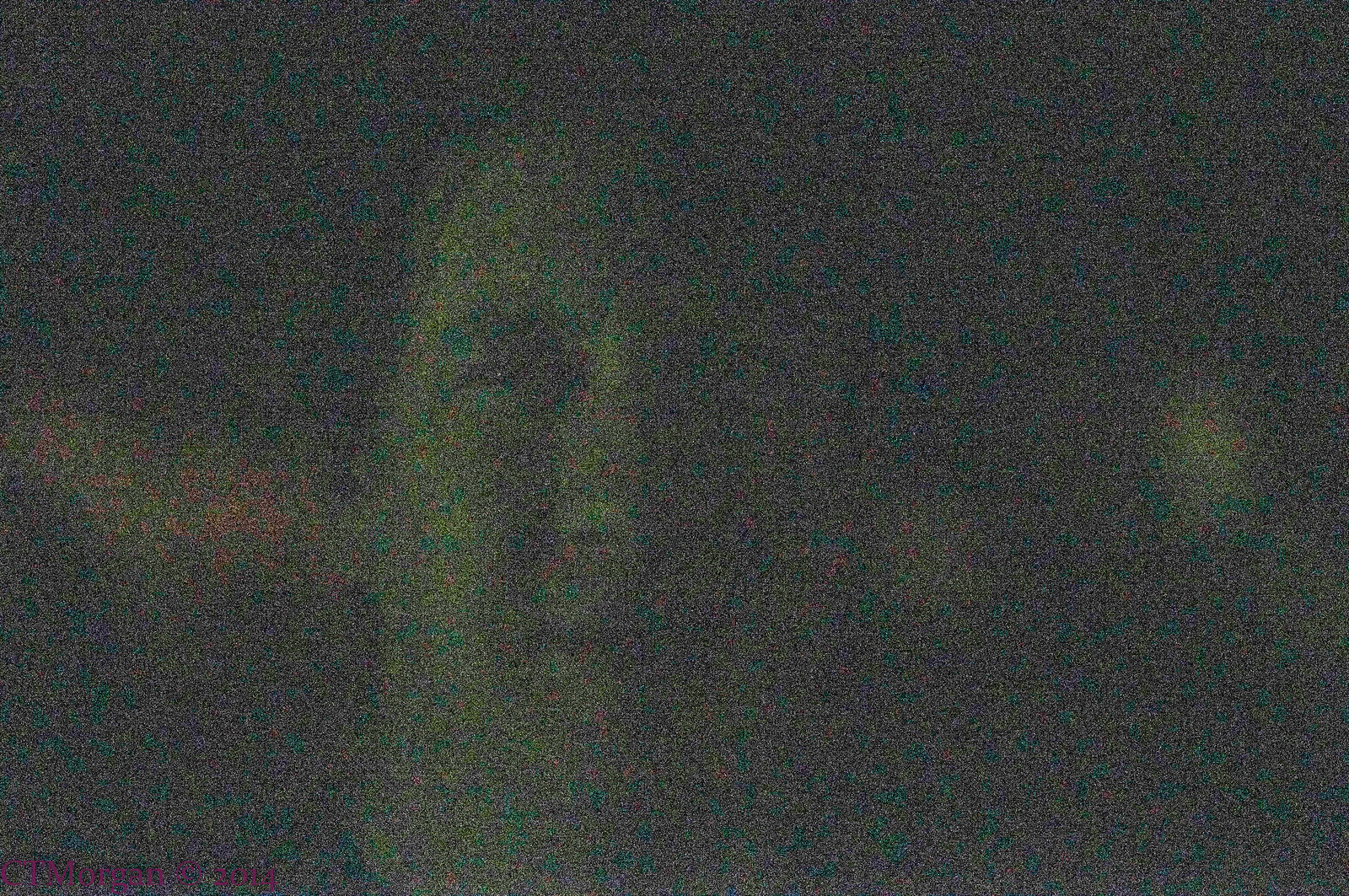The photograph depicts a man's face, captured in an extreme close-up, slightly left of center in a horizontal rectangular frame. The man's complexion is light, and he appears to be staring directly at the viewer with squinty eyes. His eyes and mouth, which is slightly open as if he might be smiling or chuckling, are faintly visible amidst the image's significant noise and pixelation. His large nose and dark hair are just discernible, though the hair's details are obscured. He seems to be wearing a dark shirt, with only his neckline and shoulders in view. 

The image is very dark and underexposed, creating a near-black overall look, dotted with specks of green, blue, red, yellow, and some orange scattered across the entire photograph. These colored specks contribute to a highly noisy and pixelated texture, making finer details challenging to distinguish. The background is predominantly indeterminate, with black and white splotches and a touch of red. Additionally, a barely legible red text appears at the bottom left, and a yellow smudge is visible on the right side of the image.